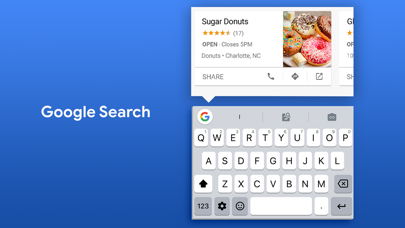The image depicts a pop-up window without any website branding. The background features a gradient from dark blue at the bottom to a lighter blue at the top. On the left side of the pop-up, "Google Search" is prominently displayed in white text within a large horizontal blue rectangle. To the right of this, there is a virtual keyboard shown with white keys and black letters, set against a gray background. 

A pop-up message overlays the keyboard, reading: "Sugar Donuts, 4.5 stars, 17 reviews, open, closes at 5 pm, Donuts, - Charlotte, North Carolina." Below this text, there’s an image featuring four colorful donuts in various shades of pink, orange, yellow, green, blue, brown, white, and dark brown. 

Small icons with labels appear beneath the image, presumably indicating options such as "Share" and "Call." At the top of the virtual keyboard, the Google "G" logo in its characteristic red, yellow, green, and blue colors appears inside a white circle on the upper left corner.

Overall, the left side of the pop-up remains mostly vacant apart from the "Google Search" note, contrasting with the more detailed content present on the right side.